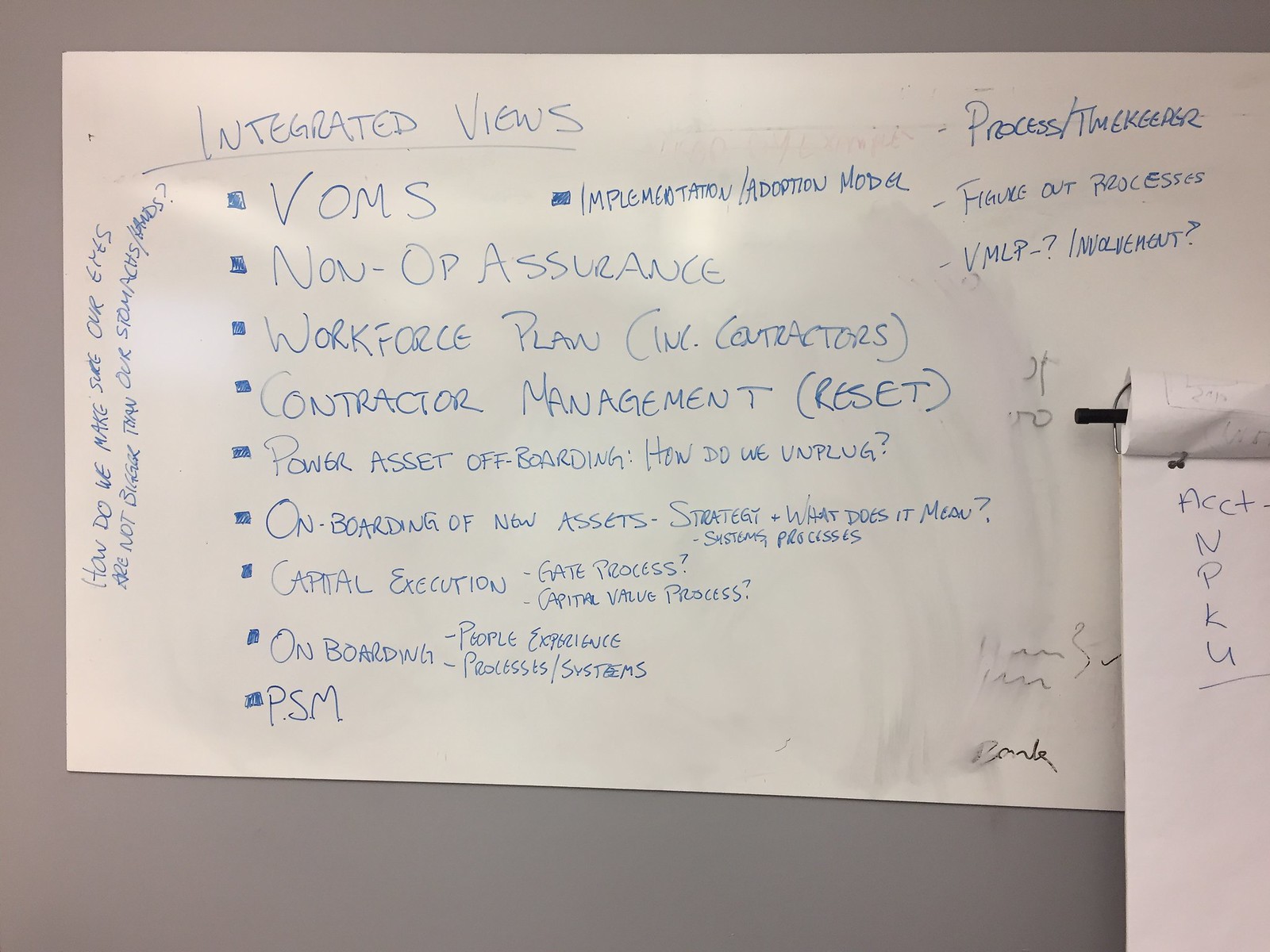The image depicts a whiteboard against a gray wall, filled with writing in blue marker. The predominant header reads "Integrated Views." Below this, there are several sections labeled as buttons, each containing detailed text. The first button includes "V-O-M-S" and "Non-Assurance Bullet Section," with terms like "Square" and "Rectangular Square Bullets." The second button outlines a "Workforce Plan," mentioning "Including Contractors, Contractor Management, Reset, Power Asset Offboarding," and "How do we Unplug?" It also lists processes like "Onboarding of New Assets," "Strategy," "Systems," and "Capital Execution Gate Process." The third button highlights key concepts such as "Processes, Systems, People Experience, and PSM."

Additionally, in the left-hand section, written vertically, are the words "How do we make sure our eyes are not bigger than our stomachs." In the top right corner, there is "Process/Timekeeper" and questions like "Figure Out Processes, V-M-L-P?" and "Involvement." 

In the bottom right corner of the image, a piece of paper on an easel displays the letters "A-C-C-T-N-T-L-U," written prominently. This detailed whiteboard encapsulates a broad range of topics and processes that seem crucial for operational planning and management.